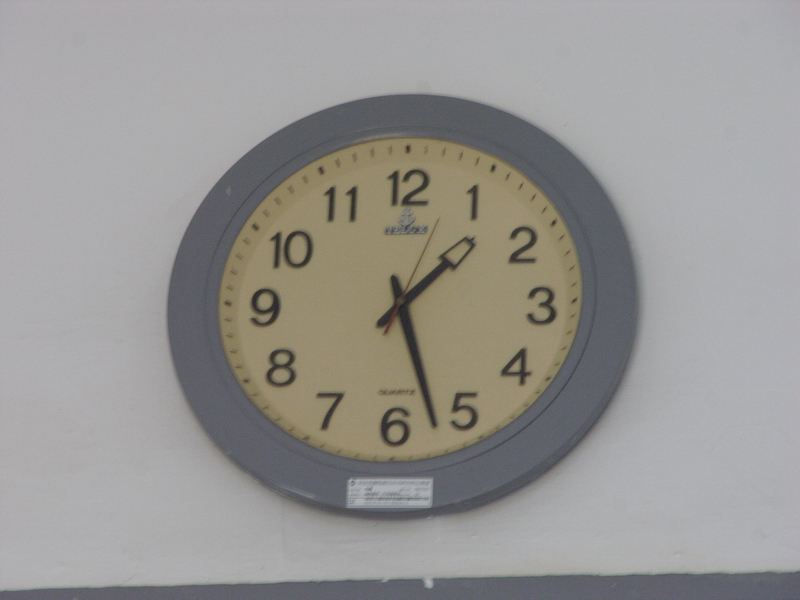This close-up horizontal image features a wall clock captured under low-light conditions, resulting in a grainy and blurred appearance. The clock boasts a wide, gray-colored frame that encircles a classic white clock face adorned with black Arial-style numerals. A prominent rectangular white label is situated at the bottom of the frame. The clock appears to have a quartz movement, with the manufacturer's name displayed just beneath the number 12, though it is unreadable due to the image's blurriness. The clock is equipped with three distinct hands: a black minute hand, a black hour hand with an open-angled end, and a vibrant red second hand. The time on the clock reads approximately 1:27. This setup is mounted against a plain white wall, enhancing the clock's minimalist aesthetic.